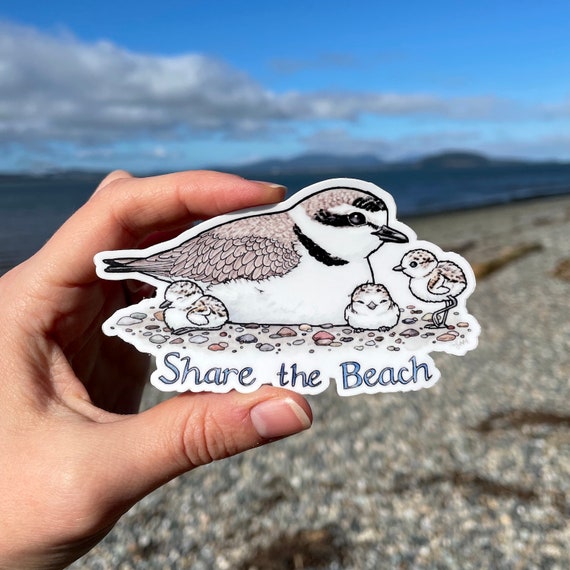This image, a square color photograph taken outdoors during the daytime, features a hand extending from the lower left-hand corner holding a white sticker between the thumb and index finger. The hand, belonging to a person of Caucasian descent, prominently displays the sticker in the center of the image. The sticker itself is a color illustration of a sandpiper-like bird with a detailed brown and beige head, black mask, and white belly. The bird is shown in profile, resting on its belly, with its beak facing the right side of the image and its tail facing the left. Surrounding the adult bird are three baby chicks, all perched on a sandy beach. Below this illustration, in italic blue cursive text, are the words "Share the Beach." In the background, which is slightly blurry, there's a scenic view of a beach with a pebble surface at the bottom, transitioning to blue ocean waves near the horizon, and culminating in a beautiful blue sky with white clouds. The right-hand side of the sky is particularly vivid, creating a picturesque and serene backdrop for the foreground sticker illustration.